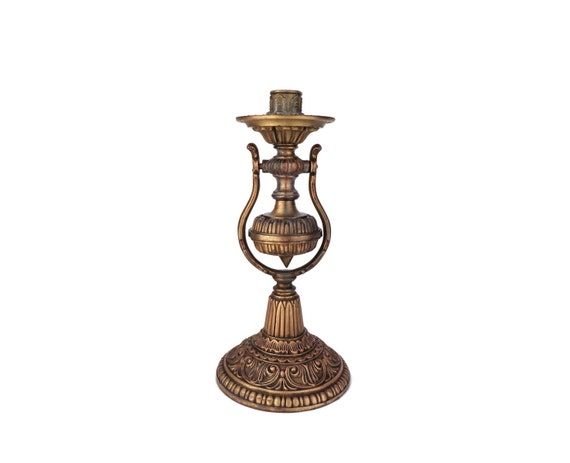This detailed photographic image features an antique candle holder set against a white background. Made of polished brass, the candle holder exhibits an intricate and ornate design. The round, wide base is adorned with elaborate scrollwork and decorative fluting, featuring patterns that resemble wings or the number nine with central dots. From the base, the structure tapers upward into a curved neck, which is accentuated by a decorative band resembling an inverted U-shape. This band supports an upper section that mimics the base's intricate detailing but on a smaller scale, culminating in another cylindrical segment. This final section flares slightly outward, designed to hold a candle. The antique piece shows black etching between its brass designs, indicating a well-maintained but aged beauty, suggesting high craftsmanship and historical value. Despite some ambiguities about its precise function, the absence of a candle in the holder and the detailed craftsmanship point convincingly to its use as an elegant candle holder.